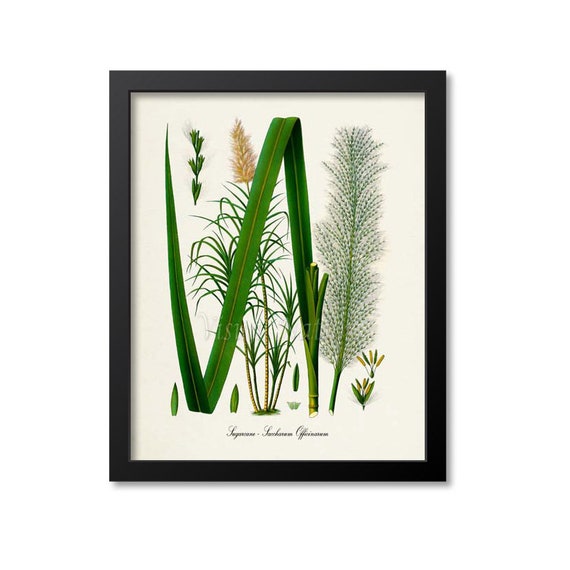The image is a detailed botanical print encased in a thick black frame, set against a white background with a vertical alignment. The artwork features a variety of plant parts in fine, either painted or drawn details, primarily in green hues. Dominating the composition is a tall plant with a green stem that rises and falls, accompanied by bushy leaves and a prominent, fuzzy cone-shaped flower partly concealed by a large blade of grass. Smaller leaves and grass-like elements are interspersed throughout, with one notably tall, feather-like structure on the right which draws attention with its delicate form. The print captures various stages of the plant's life cycle, including its seed, budding, and drying phases as the seasons change. Underneath the intricate illustrations, there is a label with small, black cursive writing, which is unfortunately too blurry to decipher but likely names the depicted plants.